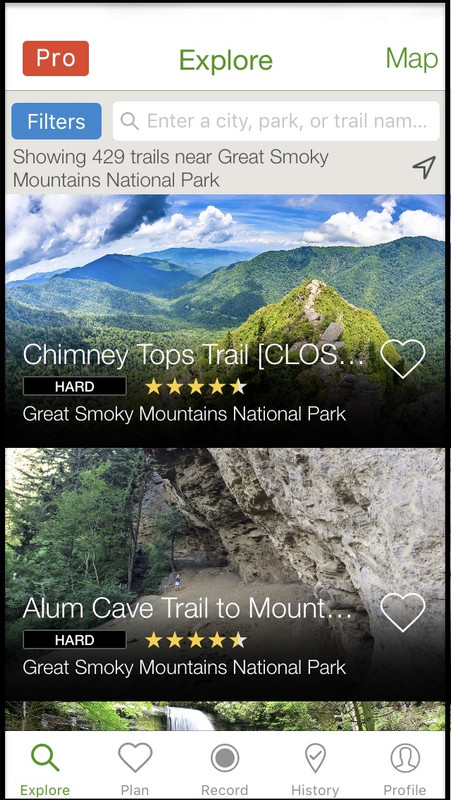The image is a vertical rectangular screenshot from a travel or tourist app. At the top, there's a horizontal white banner featuring a small red button on the left labeled "PRO" in white text, and a blue button on the right labeled "FILTERS" in white text. Adjacent to these buttons is a search bar for typing.

Directly below the banner, the app indicates it is showing 429 trails near Great Smoky Mountains National Park. Below this information are two images of trails. The first image features the Chimney Tops Trail, described as "hard" with a rating of 4.5 stars, located in Great Smoky Mountains National Park. The second image shows a large rock formation with surrounding trees, representing the Alum Cave Trail to Mount LeConte, also labeled as "hard" with a 4.5-star rating, and situated within the same national park.

At the bottom of the screen is another horizontal white banner with five icons labeled Explore, Plan, Record, History, and Profile.